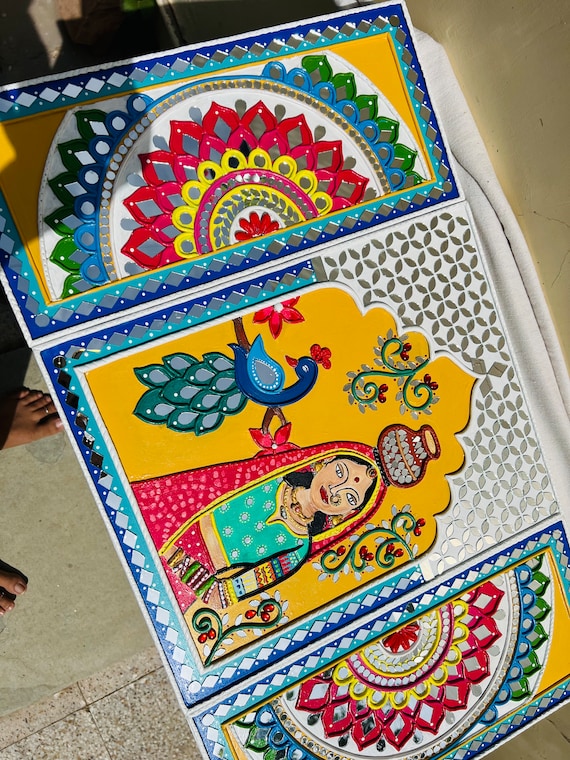The image is a photograph of a detailed piece of Indian artwork divided into three panels, likely intended to be displayed together. The central panel depicts an Indian woman, possibly a deity, adorned in a green outfit with colorful sleeves and a red robe featuring red and pink dots. She balances a clay pot on her head and is accompanied by a blue peacock on her left. The artwork's background is vibrant, utilizing a palette that includes green, light blue, red, pink, yellow, beige, orange, white, gray, and black. The two side panels appear to be decorative elements, each illustrating half of a mandala pattern with floral and repetitive designs. The panels seem to be crafted on a surface that resembles a mineral panel, which might be intended for hanging. The artwork is rich in cultural motifs and colors, creating a cohesive and lively composition. Additionally, the photograph includes a person's feet, adding an element of human interaction to the scene.